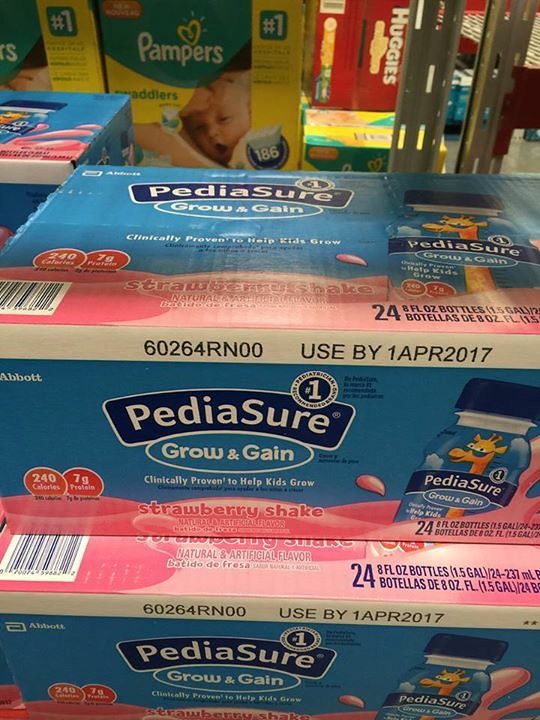In this image, large boxes of Pediasure are prominently stacked in the foreground on the Groceries 4 aisle. These boxes feature a distinct design, with blue tops, pink bottoms, and a matching blue and pink pattern on the sides. The lettering on the boxes reads "Pediasure Grow and Gain" in blue and "Strawberry Shake" in pink. The aisle itself has see-through shelves, allowing for visibility of items on the opposite side. Through the shelves in the background, a green and yellow box of Pampers diapers can be seen, and further back, a red box of Huggies diapers is also visible.